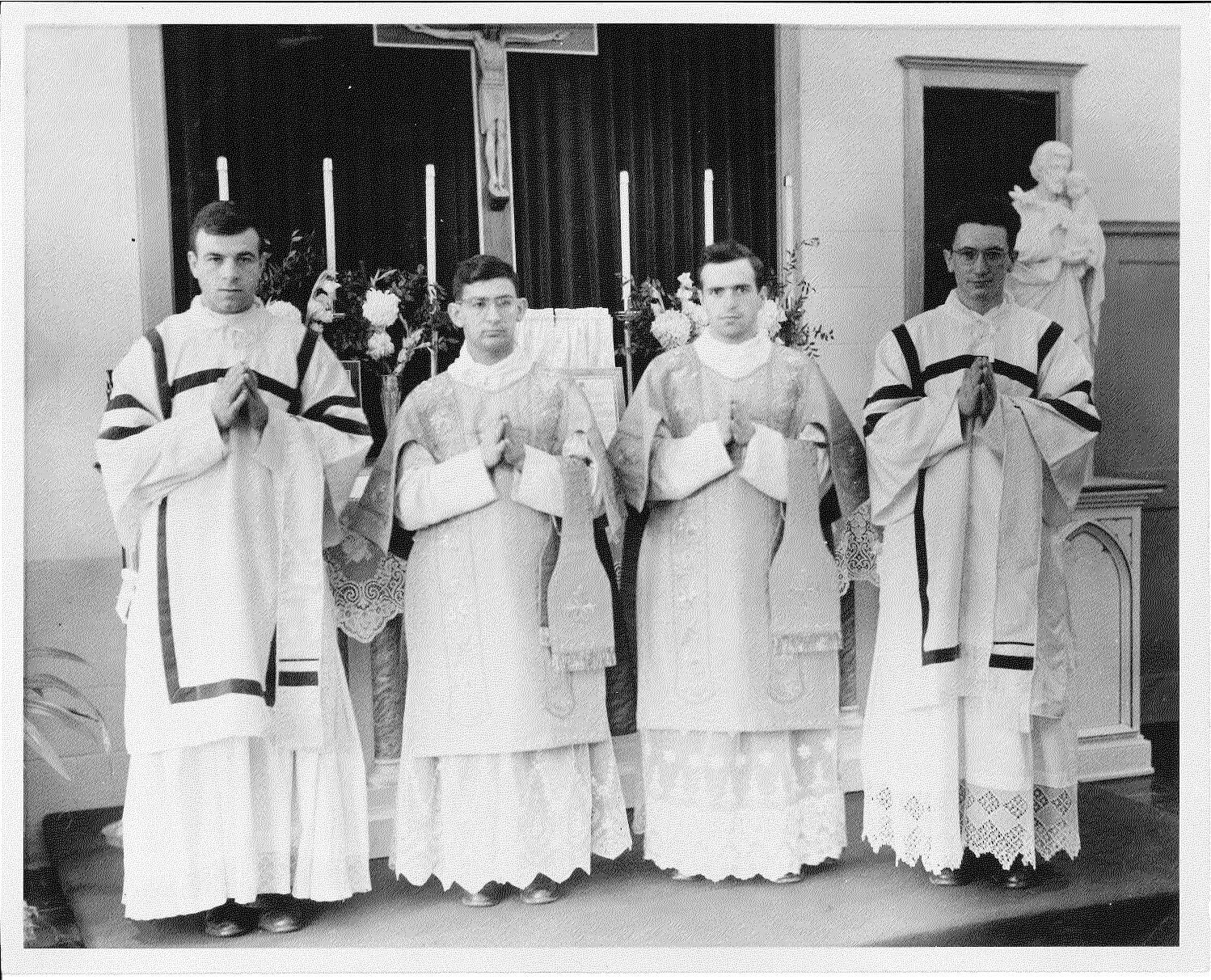This black-and-white photograph presents a solemn moment inside a church, marked by a grainy, narrow white border around its square frame. Central to the image are four youthful priests, standing on a wooden platform, each with hands clasped in a prayer-like posture. They are arranged neatly from left to right. The two priests on the ends, noticeable by their short dark hair and glasses, wear white robes adorned with distinct black outlines. They are slightly taller than the two central priests, who also wear traditional white robes but with less intricate detailing.

Above them looms a significant altar piece: a cross bearing an effigy of Christ, set against a backdrop of a long black curtain. The scene is enriched with details of church accouterments, including three unlit candles on either side of the cross, adding to the gravity of the setting. The background reveals the church interior further, showing white walls with a doorway on the right side. Completing the tranquil ambiance, a statue of a man holding a baby can be seen on the right, safeguarding the sacred environment in which these clergymen stand.